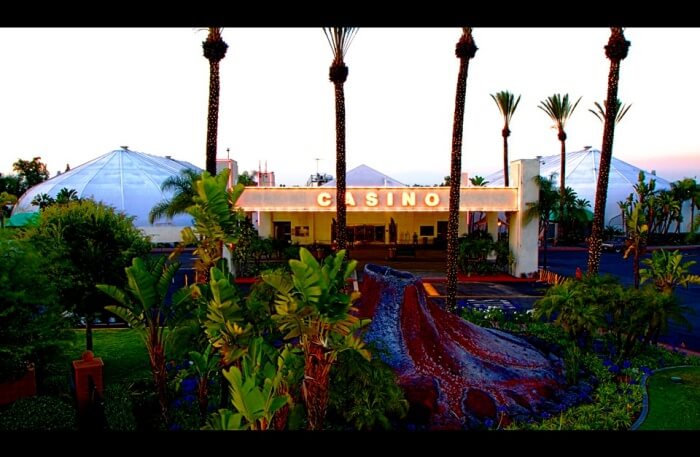The image appears to be a colorful and somewhat abstract painting of a scene featuring a small, single-story building labeled "CASINO" in off-white letters on an orangey-brown backdrop. The casino building, placed in the background, has a tan hue and features a small main entrance. The art style seems to lack fine details, favoring a blurred effect typical of oil or watercolor paintings.

In the foreground, the viewer can see a variety of trees, dominated by six palm trees—four prominently in the front and two larger ones further back. Surrounding these are other vegetative trees, adding to the lush greenery of the scene. The landscaping appears well-manicured, with vibrant green grass and sculpted gardens that enhance the painting's colorful aesthetic.

Cutting through the center of the image, from the casino towards the viewer, is a red and blue element that could be interpreted as either a waterway or a stylized path. The foreground also features what looks like a rock formation, perhaps representing a fake volcano with red and blue coloring. Additionally, there appears to be a section of blue on the ground that might suggest water or another landscaped feature.

In the very background, beyond the casino, there are more structures that add to the scene's complexity. On the left side, a dome-shaped building is visible, while to the right and further back, another dome and a pyramid-like structure can be seen. These elements, combined with a couple of rectangular buildings higher up behind the casino, create an intriguing and layered backdrop.

Overall, the painting combines natural elements with man-made structures in a visually striking and imaginative composition.